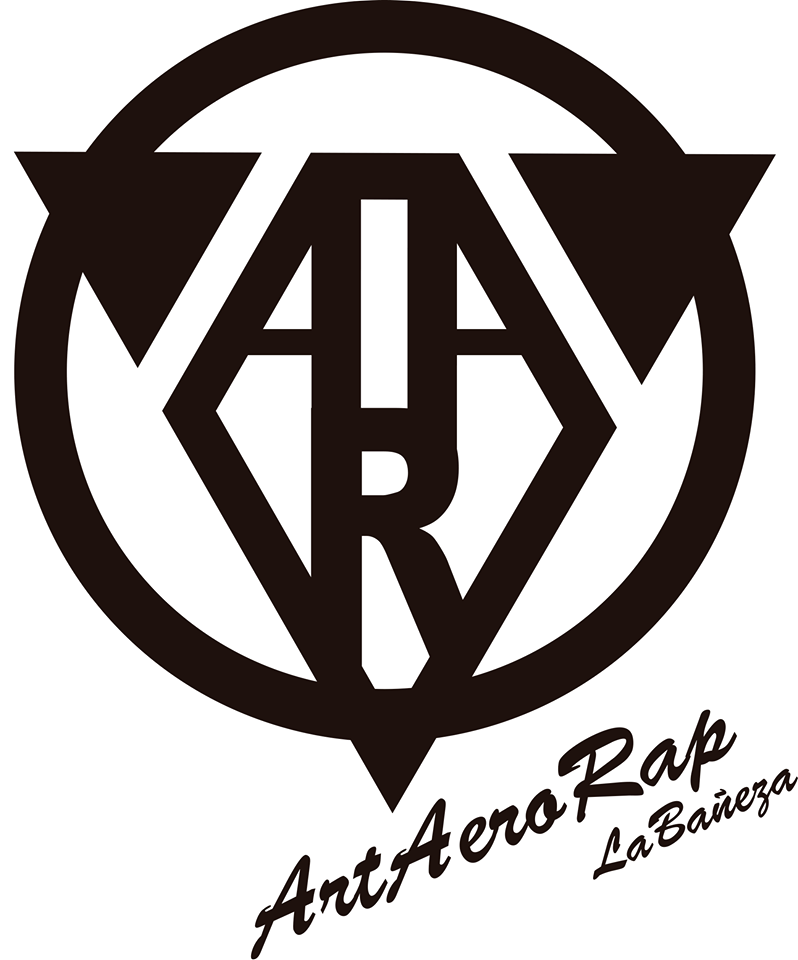The image is a monochromatic logo prominently featuring a black circle with intricate white detailing. At the base of the logo, there is text in black letters that reads "Art-Era-Rap-La-Bain-Ega La-Bain-Ega." The core design within the circle showcases two symmetrical black triangles on either side, which converge towards the center. Between them lies a diamond shape with a flat top, itself dissected by an arrangement of lines. At the bottom of the diamond is the letter 'R', from which two lines extend vertically upwards. Additional horizontal lines intersect slightly above the center of the diamond, forming smaller white triangles and a central rectangle. The overall aesthetic is modern, characterized by its geometrical precision and sleek, New Age style.